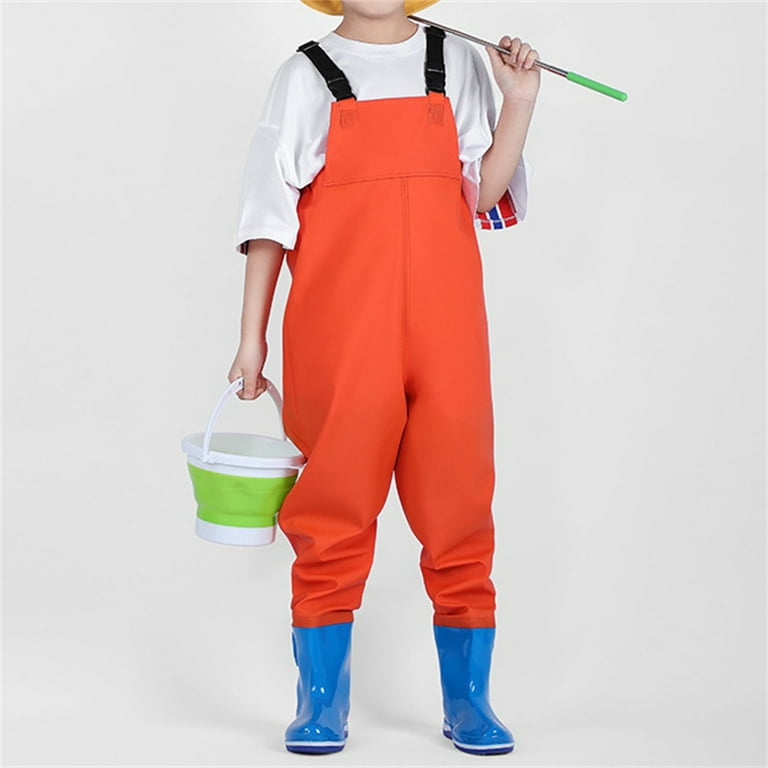In the photograph, a young boy is posing against a solid light gray background. He is dressed in orange overalls with black straps and a white t-shirt that has a red and blue stripe on the side. His outfit includes blue insulating boots that are splashed with white paint. He appears to be dressed as a painter or perhaps a young fisherman. In one hand, he holds a green and white paint bucket, while the other hand rests a fishing pole with a metallic green handle on his shoulder. Additionally, he is wearing a hat with a brim, although his face is not visible. The plain light gray backdrop emphasizes the colorful attire and objects he is holding, making them the focal point of the image.